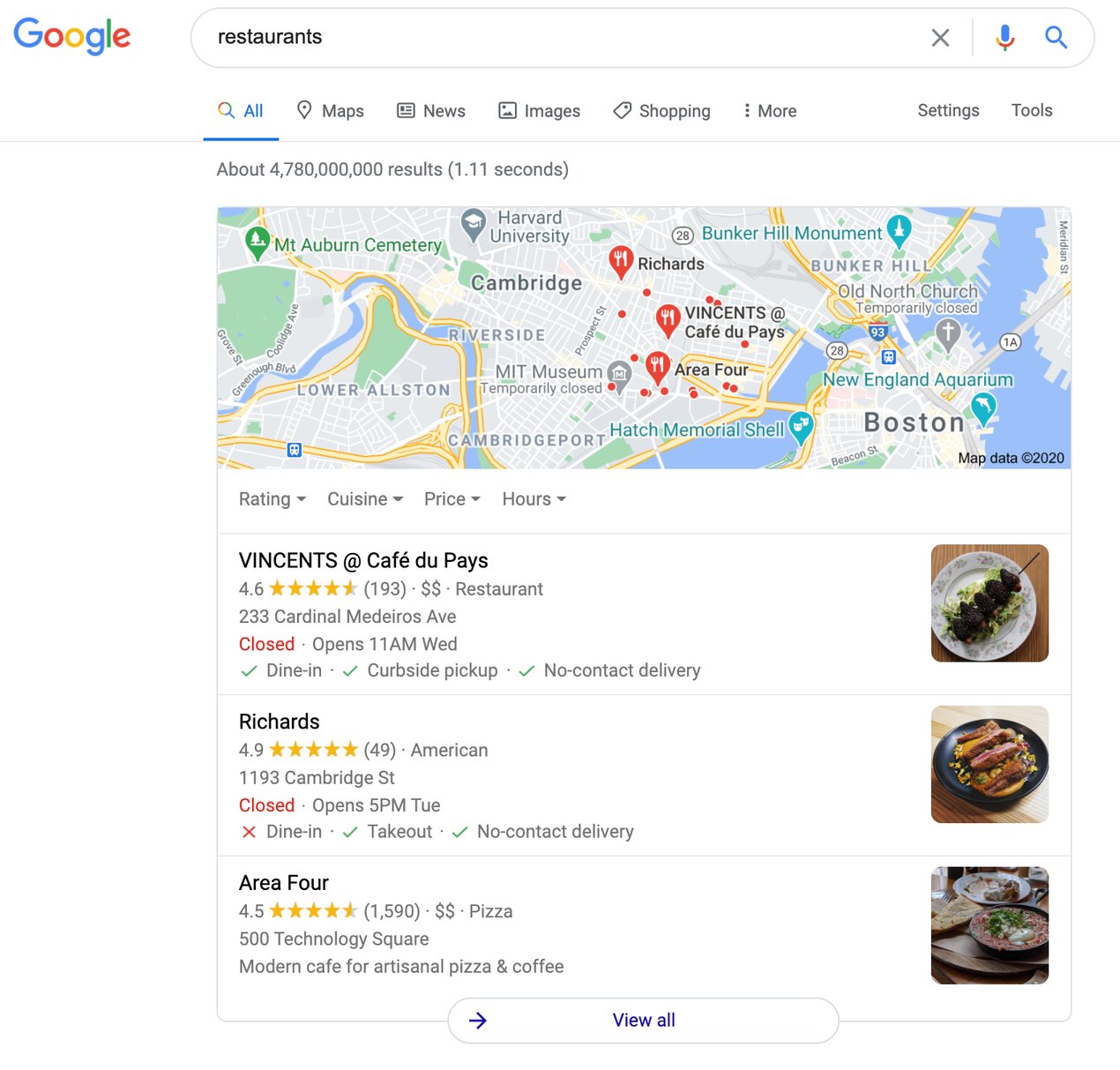This screenshot is a detailed capture of a Google search result for "restaurants," predominantly featuring a white background without defined borders. The image is in portrait orientation and shows the interface of a typical Google search page. 

In the upper left corner, the multi-colored Google logo is prominently displayed, featuring its signature colors of green, blue, red, yellow, and green in that specific order. Below the logo, there is a white search bar with the word "restaurants" entered in black text.

Directly under the search bar are filtering options for the search results, including "All," "Maps," "News," "Images," "Shopping," and more. "All" is selected and highlighted in blue with an underline, accompanied by a magnifying glass icon in Google's color scheme. Beneath these filters, the text indicates that there are about 4.78 billion results, retrieved in approximately 1.11 seconds.

A horizontal, rectangular map is displayed below this text, showing a few highlighted locations. Following the map, there is a section displaying individual restaurant listings in a white background. Each listing includes a thumbnail image on the right and corresponding restaurant information on the left.

The first listing is for "Vincent at Café des Pays," rated 4.6 stars out of 193 ratings. The second listing is for "Richards," boasting a 4.9-star rating from 49 ratings. The third listing is for "Area 4," which has 4.5 stars garnered from 1,509 ratings. Each entry provides an ample summary, including names and ratings, allowing users to quickly glean the quality and popularity of each restaurant.